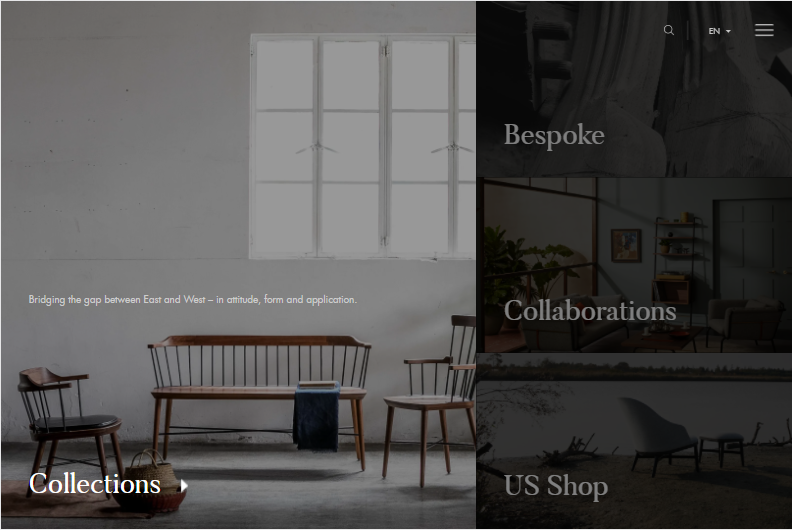The image is a screenshot from a website or app, primarily featuring a collage-like layout composed of multiple images. 

At the top right corner of the screenshot, there is a small 'burger' menu button for navigation options. To its left is a language selection dropdown currently set to English (EN), indicated by a downward-pointing triangle. Next to the language option is a magnifying glass icon representing the search function.

On the right-hand side of the screen, occupying about one-third of the image, there are three vertically stacked sections labeled "Bespoke," "Collaborations," and "US Shop," each accompanied by a distinct but darkened background image:
- "Bespoke" features an image that appears to be a sculpture.
- "Collaborations" displays what looks like a seating area within a home.
- "US Shop" shows a chair positioned in front of a body of water.

The remaining two-thirds of the image on the left side are dedicated to a section titled "Collections." Below this title, there is a tagline that reads, "Bridging the gap between East and West in attitude, form, and application." The background image for this section depicts a sparsely decorated room featuring large windows at the back, a wooden bench, and two wooden chairs.